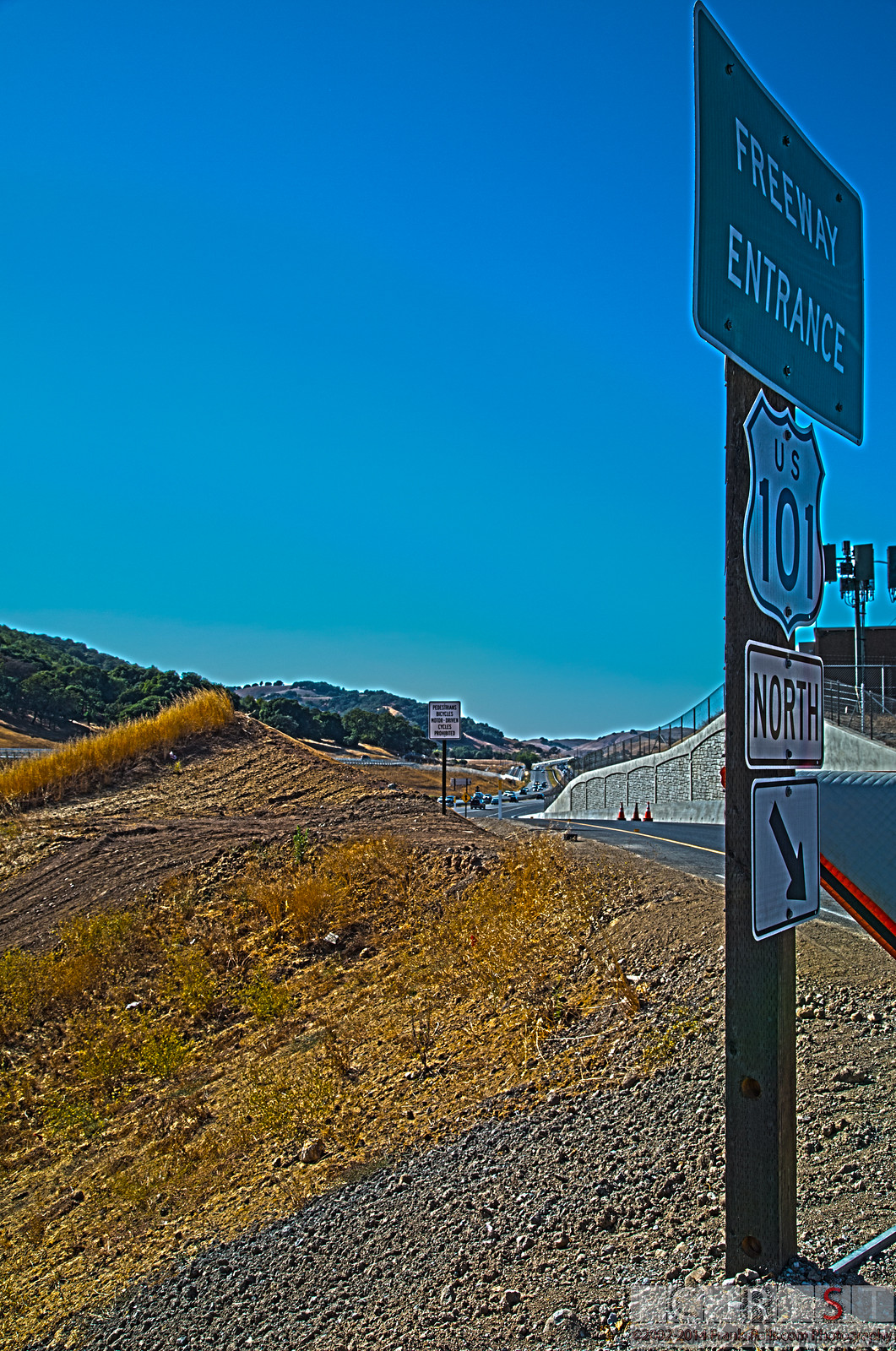In this image, there is a detailed view of a road sign cluster positioned on a gravel shoulder, framed by a sloping hill with yellow vegetation and dirt. The central sign is mounted on a dark pole and is seen against the backdrop of a blue sky and green hills. The sequence of signs from top to bottom includes a long rectangular green sign with white letters stating "Freeway Entrance," followed by a U.S. 101 Highway shield. Below this, a white sign with black lettering indicates "North," accompanied by a square white sign with a black arrow pointing down to the right, directing traffic towards the freeway entrance. To the right of the image, there is a single-lane road with traffic cones and a white wall on its side, leading up to the entrance ramp. In the background, partly obscured, there's another sign possibly cautioning against driving on the shoulder. The setting appears to be outdoors during the middle of the day.